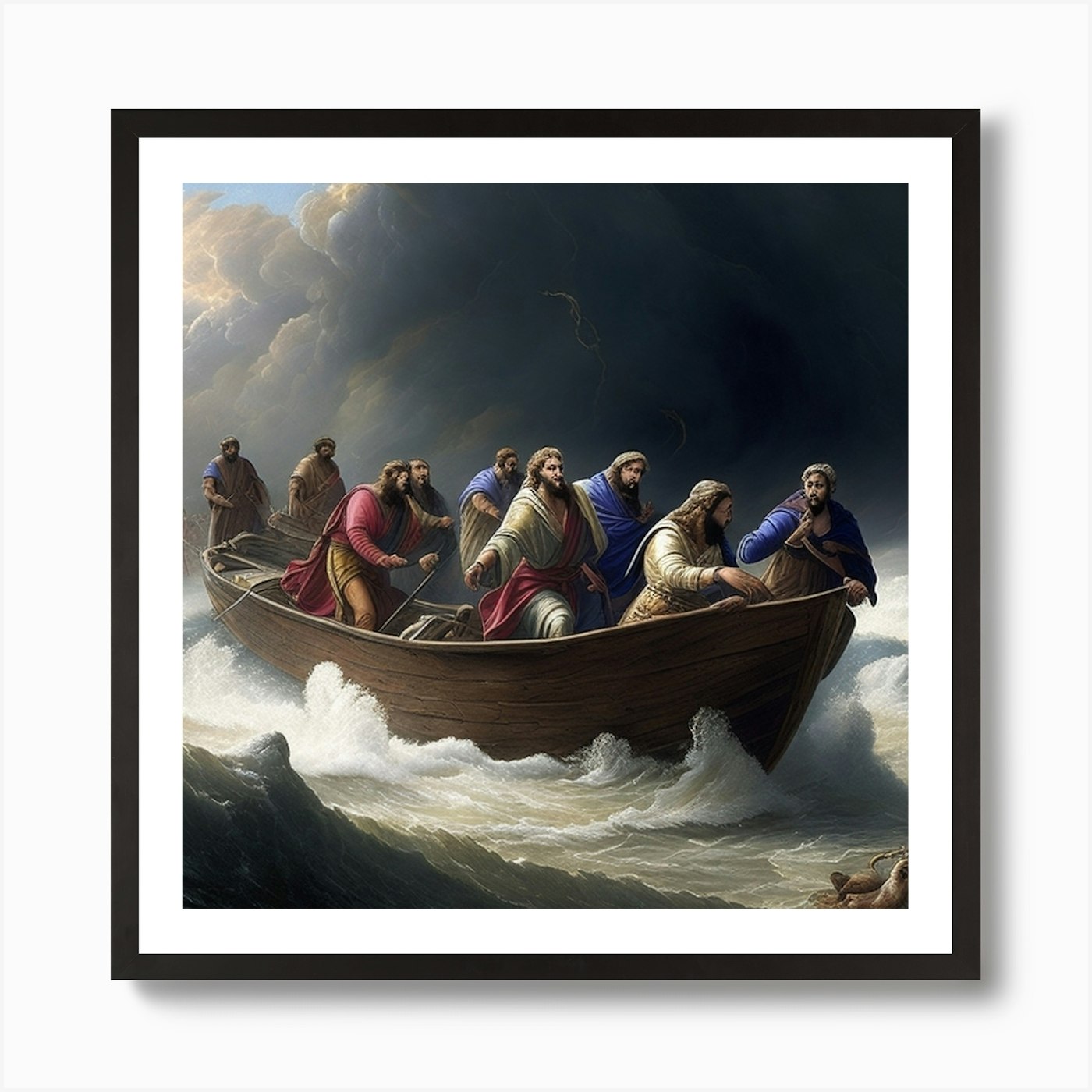The artwork in the image is a vibrant, color print, framed in black, depicting a biblical scene set during a thunderous storm. The composition shows Jesus and several men, presumably his disciples, in a large, wooden boat tossed by rough, tumultuous waves. The boat is small yet large enough to carry multiple figures, nine in total, scattered across what appears to be two interconnected boats. Jesus, identifiable by his white robe and red sash, stands out amidst the chaos, surrounded by companions in varied robes of blue, red, and beige tones. Their long hair and flowing garments evoke the historical ambiance of Biblical times.

The backdrop features dark, brooding clouds with hints of lightning illuminating the stormy sky, contributing to the dramatic atmosphere. The only hint of calm is a sliver of blue sky in the upper left corner of the image. The scene is encased in a black frame with a white mat, all set against a stark white wall, enhancing the striking contrast of the artwork.